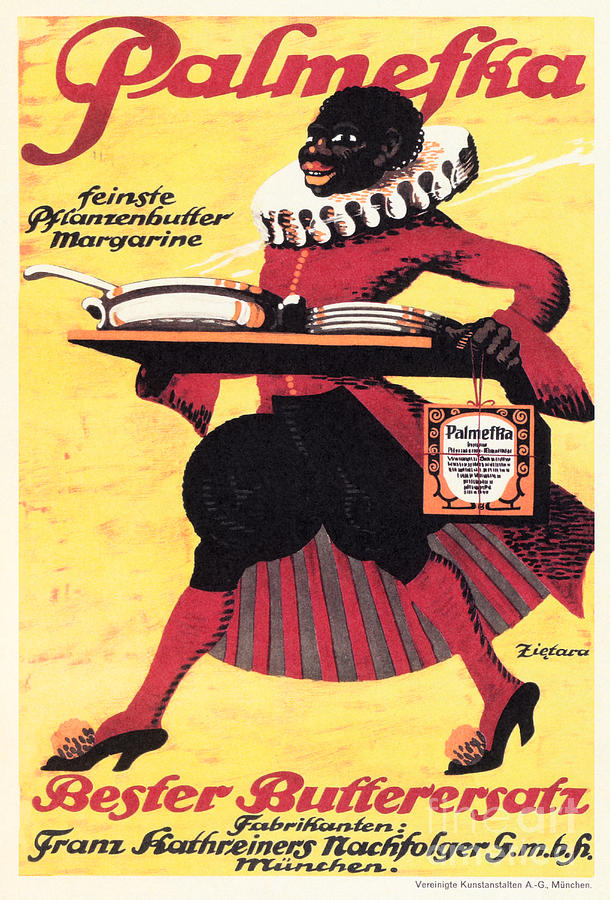The image is a vintage advertisement poster featuring a bright yellow background with a light pink border. At the top, in bold red lettering, it reads "Palmefka." Below this, in black text, it says "Feinster Pfluffen Butter Margarine," indicating it's an ad for a type of butter or margarine. The central figure is a black woman dressed in an elaborate, old-fashioned outfit. She has a very dark face and short black hair, and her attire includes a massive ruffled collar, a tight bodice, tight sleeves with large cuffs, bloomers, and an elegant coat with knee-length tails lined in gray and pink stripes. She wears red stockings with black stripes up the back and high-heeled black shoes. She is holding a serving platter with plates and a white skillet, and she also holds a patterned square box wrapped in red threads. At the bottom of the poster, there are various inscriptions in red and black, including the words "Bester Butterstar," and additional details like "Catherine Nespolgar GmbH, Munchen," and "Vereniginte Konstantin A.G., Munches," suggesting a German origin.